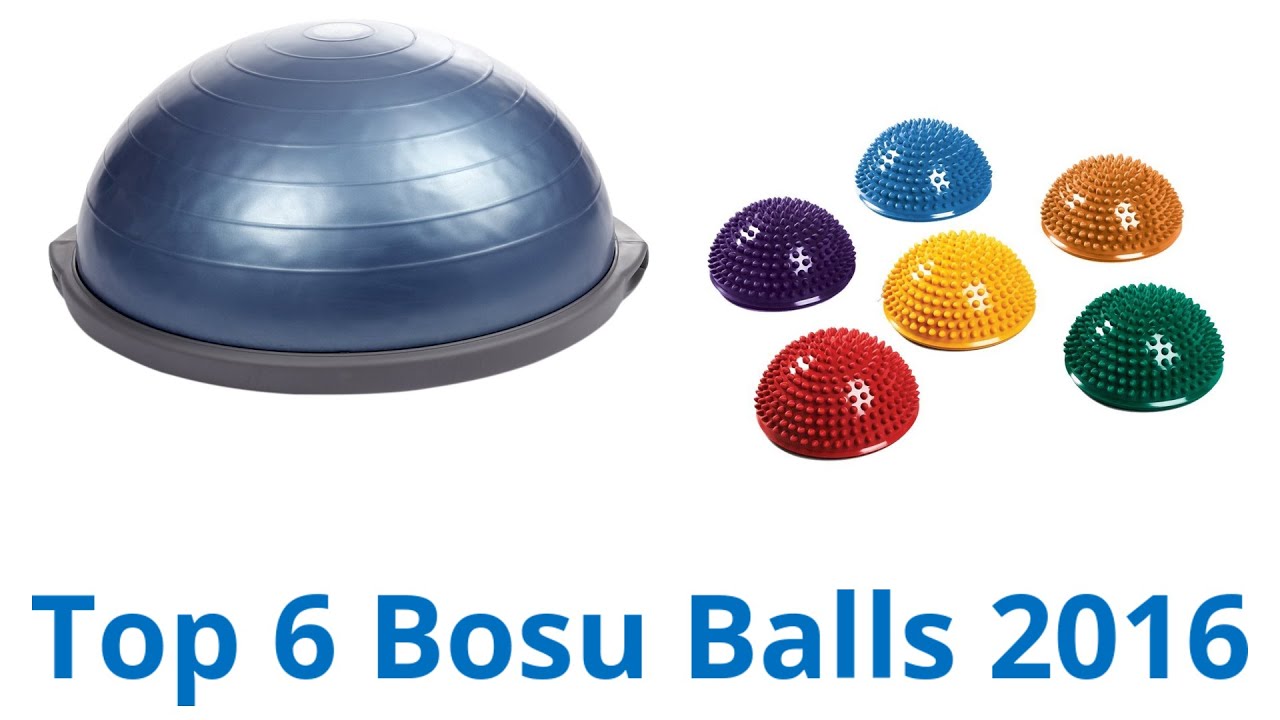This professionally-taken photograph appears to be an advert for the top six BOSU balls of 2016. Dominating the left-hand side of the image is a large silver-gray BOSU ball, placed on a black base. On the right-hand side, six smaller, spiky exercise balls, possibly made of plastic, are grouped together. These balls are arranged with five forming a circle and one in the center, featuring the colors purple, light blue, brown, green, red, and yellow. Below the balls, the text "Top 6 BOSU Balls 2016" is prominently displayed in blue letters. The image has a clean, white background and includes no additional elements or people, suggesting it might have been sourced from a blog rather than a polished advertising campaign.